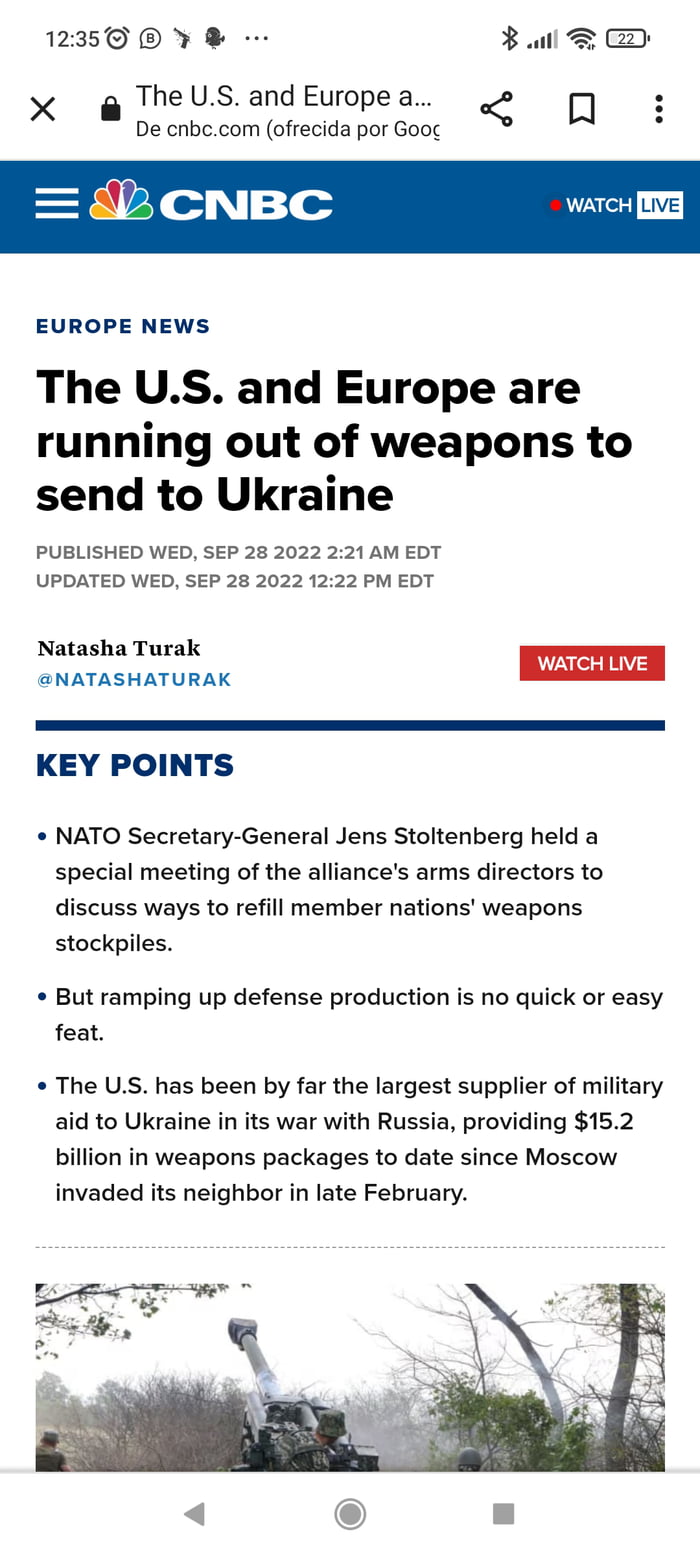This detailed caption describes an image taken from a CNBC article being read on a mobile phone:

---

The image captures a screen from a CNBC article viewed on a smartphone. The distinctive CNBC logo, resembling colorful turkey feathers in a vibrant rainbow hue, adds a striking backdrop. Prominently placed is a red circular icon with the text "Watch Live." Below the icon, the heading reads "Europe News," followed by the headline: "The U.S. and Europe are running out of weapons to send to Ukraine." The article was initially published on Wednesday, September 28, 2022, at 2:21 a.m., and includes an update timestamp. 

On the right side of the screen, there's a rectangular prompt labeled "Watch Live." The left side features the byline "Natasha Turek @NatashaTurek." The section "Key Points" follows, each point marked by bullet points:

1. NATO Secretary General Jens Stoltenberg held a special meeting with the alliance's arms directors to discuss how to replenish member nations' depleted weapons stockpiles amid ongoing conflict.
2. Ramping up defense production to meet these needs is identified as a complex and challenging task.
3. The U.S. has significantly contributed to Ukraine's military aid, supplying $15.2 billion in weapons since Russia's invasion in late February.

A related image appears at the bottom of the screen, further illustrating the article's content.